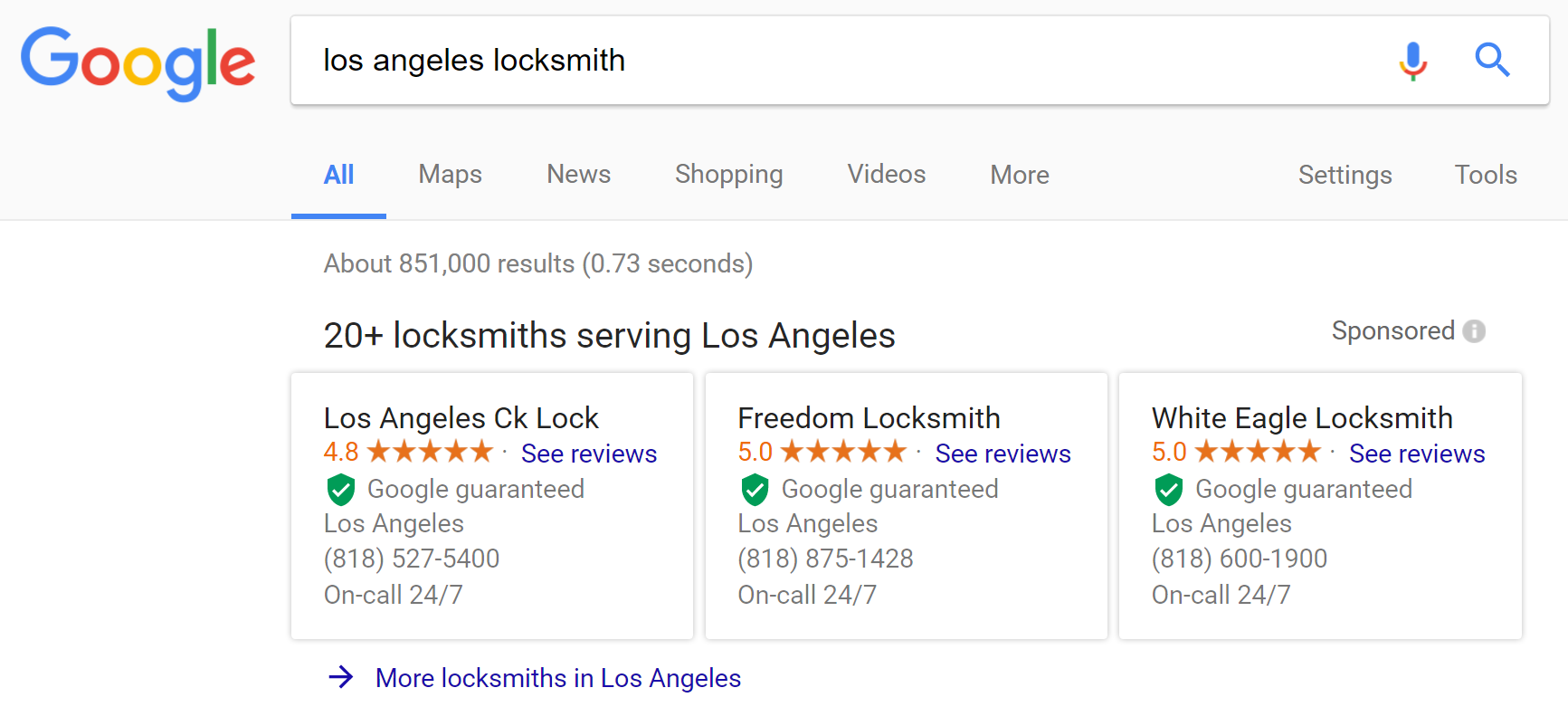This screenshot, taken from a desktop or laptop computer, displays results from a Google search query. Against a white background with a light grey header, the Google logo is prominently displayed. In the search bar, black text reads "Los Angeles locksmith," accompanied by a microphone icon and a magnifying glass symbol for search functionality.

Below the search bar, a navigation menu features tabs labeled "All," "Maps," "News," "Shopping," "Videos," "More," "Settings," and "Tools." Directly beneath this menu, the search results statistics are shown: approximately 851,000 results found in 0.73 seconds. A highlighted section reports "20+ locksmiths serving Los Angeles," immediately followed by the term "Sponsored" with an accompanying information icon.

The primary search results are listed below this section, beginning with "Los Angeles CK Lock," which has a 4.8-star rating and further contact details. Adjacent listings include "Freedom Locksmith" and "White Eagle Locksmith," each featuring similar rating information. Additional options to search for more locksmiths in Los Angeles are provided at the bottom of the results.

This descriptive caption captures the detailed layout and specific elements visible in the screenshot of the Google search results page for "Los Angeles locksmith."